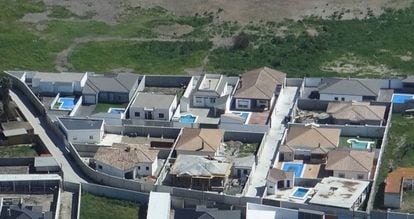This aerial photo, taken during the day, captures a detailed view of a small, densely-packed neighborhood. The image reveals a collection of houses, each enclosed by individual fences that create distinct square sections. Most of the houses are one-story structures with flat or slightly arched roofs, painted predominantly white or dark colors with some tan roofs. Accompanying each house is a secondary structure, possibly a garage or an additional small dwelling. Several properties feature small backyard pools, adding a touch of blue amidst the neutral tones. A main road winds from the middle left of the photo, curving downwards and stretching to the bottom right, flanked by walls on either side. The neighborhood occupies the lower two-thirds of the photo, with the upper third showing a grassy field interspersed with weeds and dirt, and sections of sandy terrain beyond the neighborhood’s fences and walls. There’s also a narrow walkway running behind the houses. The overall scene lacks text or other indicators that could suggest a specific location.